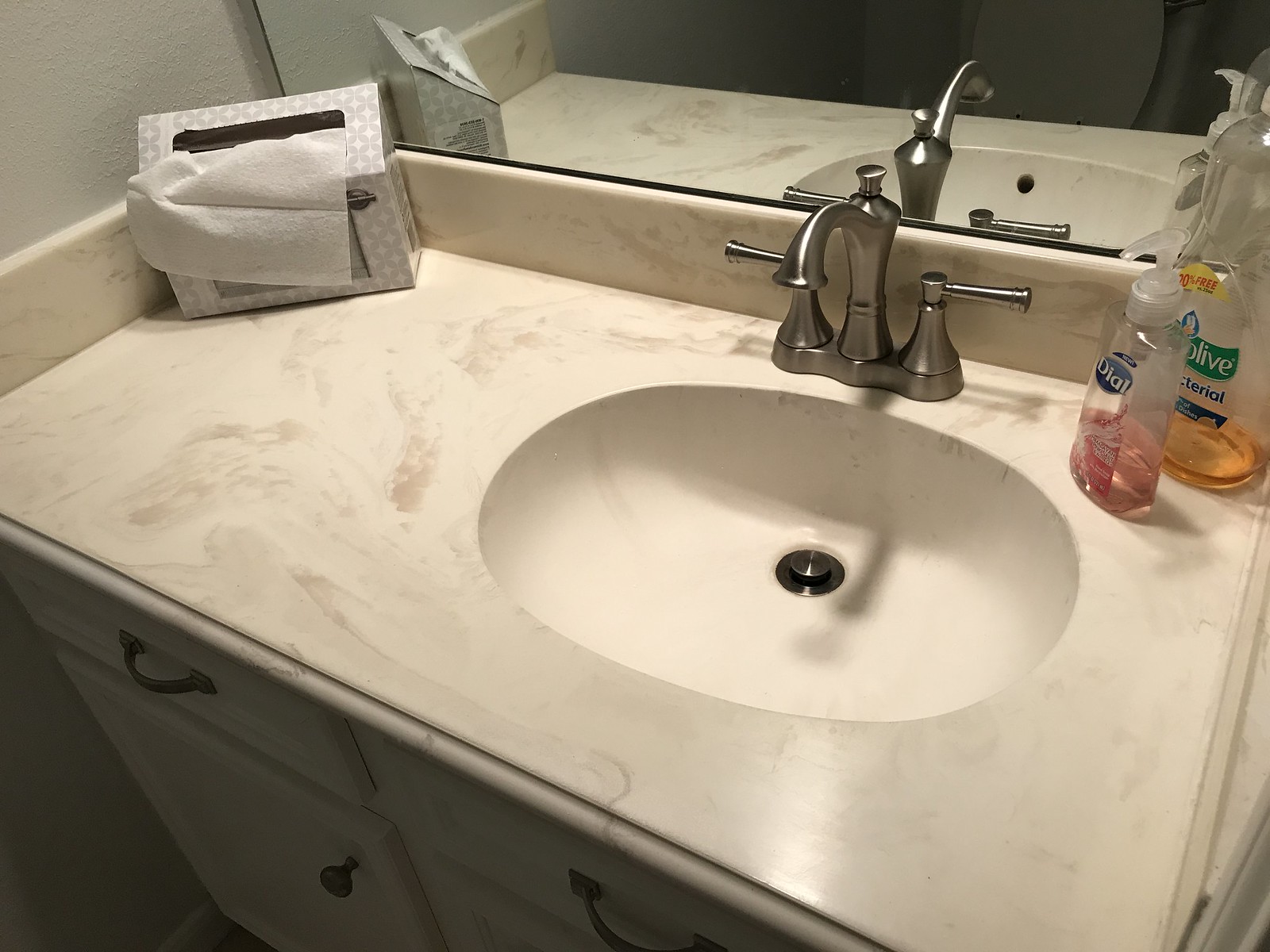This photograph captures a detailed view of a bathroom sink set against a white, stucco-textured wall. The sink is beautifully inset into a countertop that features a luxurious white and gray marble pattern. On the left side of the sink, a box of tissues stands with one tissue delicately folded over the top, adding a touch of practicality and elegance. The sink itself is an oval basin with sophisticated, pewter-colored fixtures, including two handles and a sleek faucet. To the right of the sink, two bottles of liquid soap are placed next to each other. The shorter bottle, featuring a pump top labeled "Dial," contains a light pink liquid soap that is approximately one-fourth full. The taller bottle, partially obscured, displays fragments of text including "olive" and either "bacterial" or "antibacterial," and holds a small amount of dark yellow liquid at its base. Behind the sink, a mirror reflects the tissue box, the sink, its fixtures, and the soap bottles, adding depth and continuity to the scene.